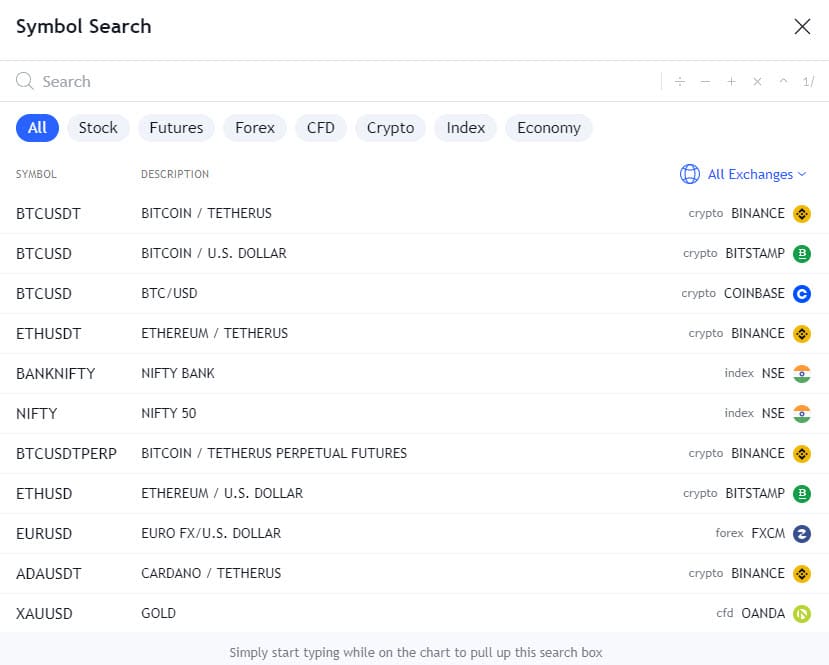This image is a screenshot of an application or website interface for cryptocurrency trading or monitoring. 

The interface features a clean white background with primarily black and gray text elements. In the top-left corner, a header labeled "Symbol Search" is prominently displayed. On the upper-right corner of the interface, an 'X' icon can be seen, presumably to close the current window or dialog.

Just below this is a search bar equipped with a magnifying glass icon to its left, indicating its function for text input. To the right of this search bar are several mathematical operation symbols: division (÷), subtraction (−), addition (+), multiplication (×), an upward-pointing caret (^), and a fraction symbol (⁄).

Below this search bar, a row of selectable menu items is presented. These menu items include categories such as "All," "Stock," "Futures," "Forex," "CFD," "Crypto," "Index," and "Economy." Each category is encapsulated in an oval button with a gray background and black text, except for the "All" button, which is highlighted with a blue oval and gray text, indicating it is the currently selected category.

The main portion of the screenshot features several rows of cryptocurrency listings. Each row is organized under column headings labeled "Symbol," "Description," and a drop-down menu labeled "All Exchanges" on the right-hand side. This section displays various cryptocurrencies, such as Bitcoin (BTC), Ethereum (ETH), and Cardano (ADA), among others, providing detailed and categorized information useful for the user.

Overall, the interface appears streamlined and user-friendly, aimed at those involved in cryptocurrency trading or analysis.